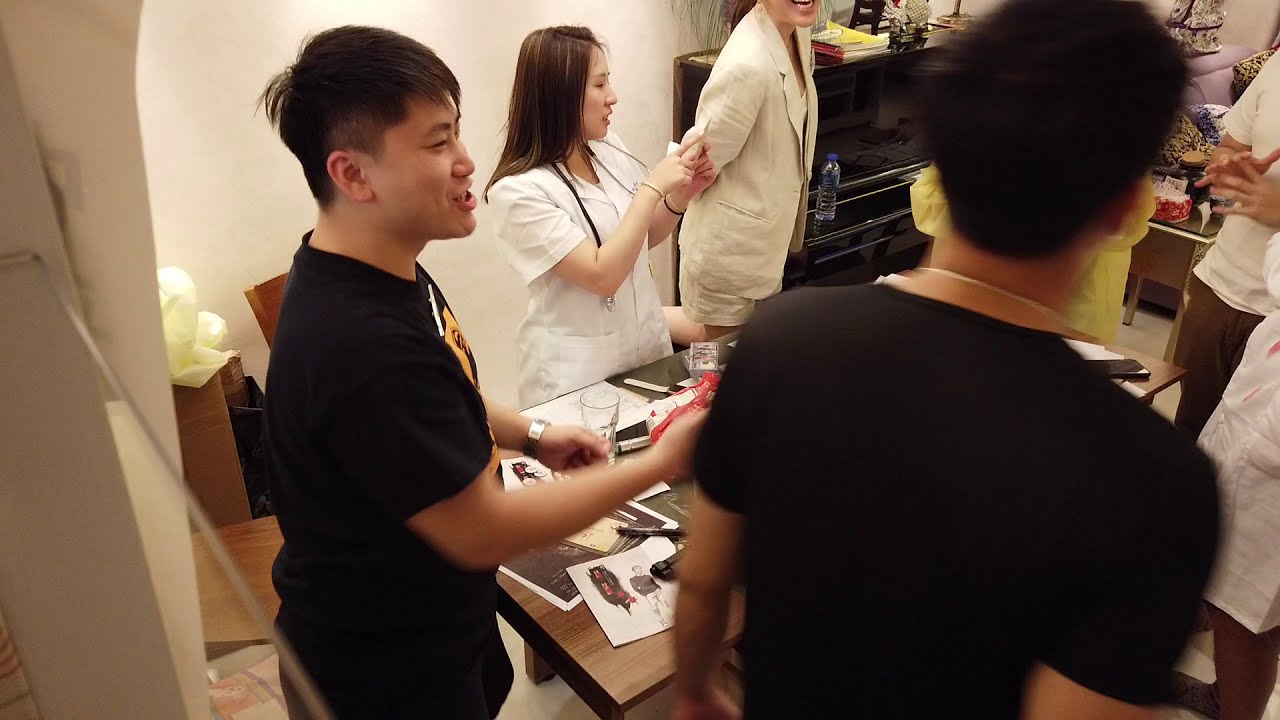The image captures a dynamic scene within a room populated by a diverse group of people, mostly of Asian descent and engaged in what appears to be a lively discussion. The setting is somewhat ambiguous, as it could be a business, school, or fashion-related environment. In the immediate foreground on the right side, a somewhat blurry figure wearing a black shirt with a white necklace or lanyard can be seen, their back turned to the camera. Next to this person stands another individual also dressed in a black t-shirt, with a glimpse of a white and yellow logo on it. Both appear to be male.

A bit further into the room, a woman dressed entirely in white captures attention; she has a stethoscope around her neck, suggesting she could be a medical professional. She has brown hair and appears to be holding something up for examination. To her right, another person in a cream-colored jacket is not only smiling but also adds to the friendly atmosphere. The crowd includes others whose faces are partially obstructed or cut off.

Central to the scene is a large brown wooden table cluttered with various papers that seem to feature fashion drawings, alongside pens and a bottle of water. This table acts as a focal point for the group, suggesting they are reviewing or discussing the contents. The overall vibe is bustling and collaborative, enriched by the detailed elements scattered throughout the room.